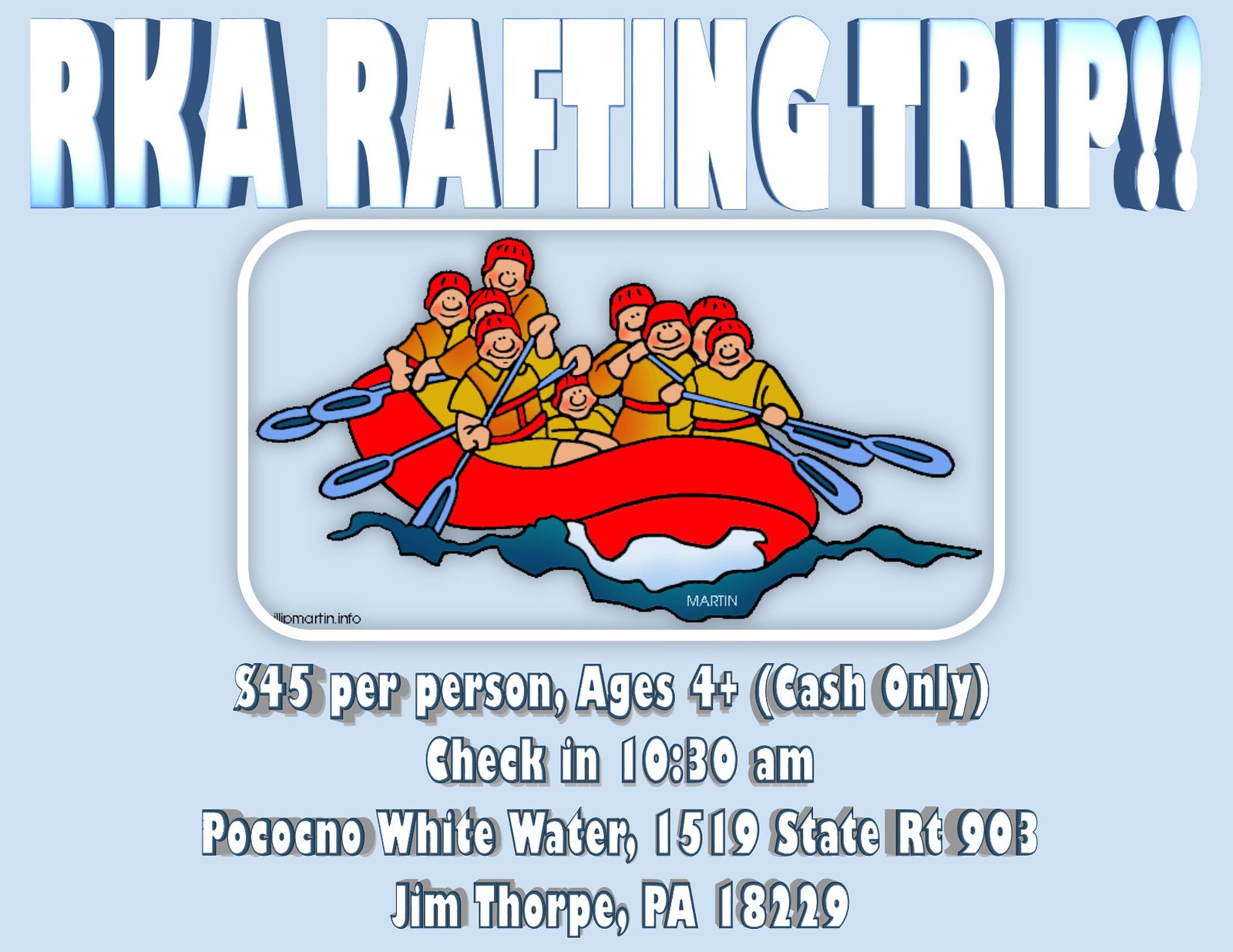The advertisement showcases an exciting rafting trip, prominently featuring bright white bubble text reading "RK Rafting Trip" at the top, set against a baby blue background. Dominating the center is a vivid clipart depiction of eight male figures dressed in life jackets, energetically paddling with blue paddles in a vibrant red inflatable raft through calm waters. Below this engaging illustration, detailed text offers essential trip information: the cost is $45 per person, for ages 4 and up, with cash-only payments accepted. Check-in is scheduled for 10:30 AM at Pocono Whitewater, located at 1519 State Road 903, Jim Thorpe, PA 18229. The overall design, with its playful color palette of blue, white, red, and orange, effectively captures the adventure and fun of the event.